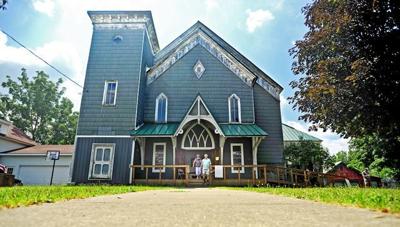The image captures a striking, tall blue farmhouse viewed from the perspective of the driveway or walkway leading up to it, making the house appear grand and imposing. The house features a distinctive tower-like section on the left side, characterized by a large, square structure that rises to nearly three stories. The exterior is painted blue with contrasting white trimmings, including an elegant arch at the front entrance. A cozy wooden deck extends across the front of the house and down one side, bordered by bright yellow-green grass. Two people stand on the front porch, adding a sense of scale to the tall, stately home. In the background, additional buildings such as houses or garages can be seen, along with a basketball hoop and a large tree to the right. The scene is set against a backdrop of clear blue skies adorned with fluffy white clouds, contributing to the overall serene and picturesque setting.